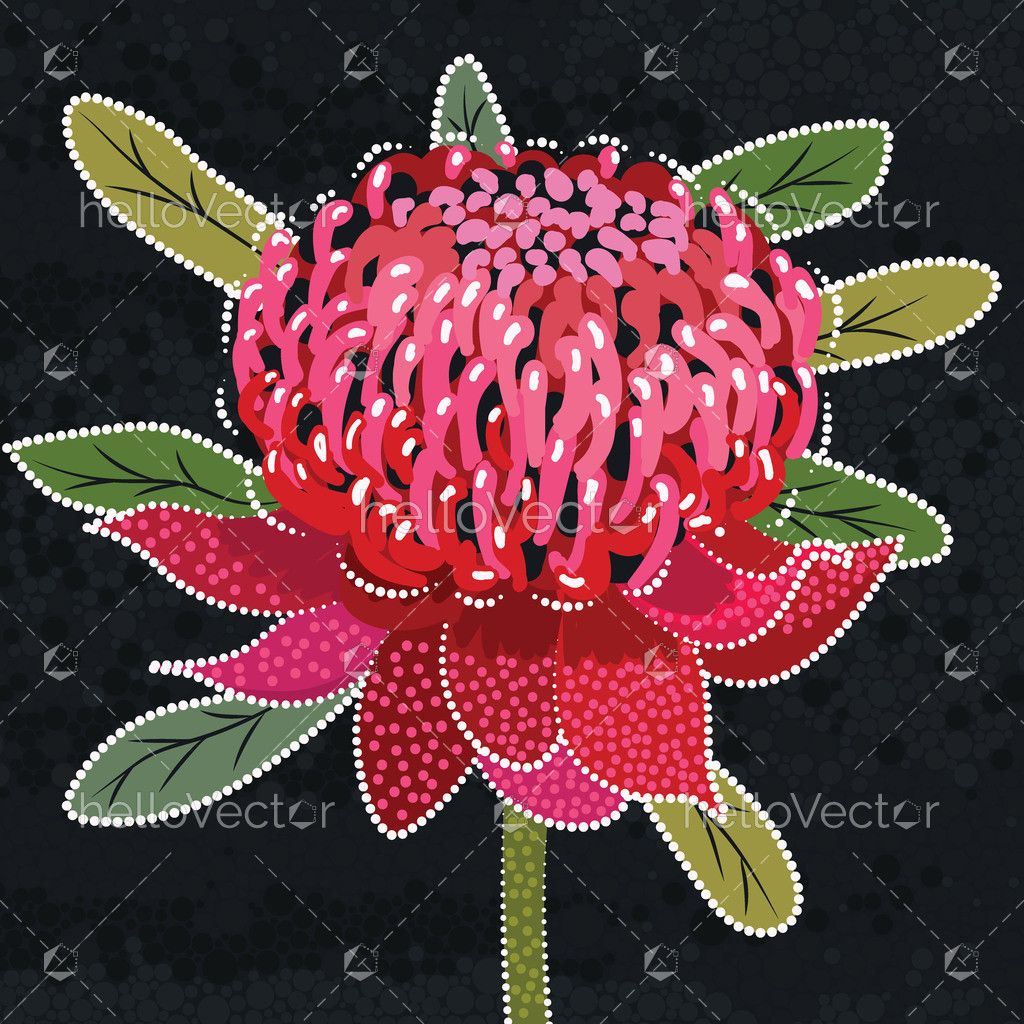This illustration depicts a highly stylized, digitally created flower from a Vector website, prominently watermarked with "Hello Vector." The flower, set against a completely black, diamond-sectioned background, features a dramatic color palette of pink, red, and purple for its rounded petals, and has additional, more conventional petals at its base. Encircling the flower are eight elongated green leaves, which are spaced apart and do not touch. The flower’s stem is a dark green, and both the flower and stem are outlined with white dots, suggesting a dot art style. The central bud of the flower, in shades of red and pink, somewhat resembles a brain in its intricate blossoming form. The entire image is composed of flat colors typical of vector graphics, providing a clean and vivid artistic representation.